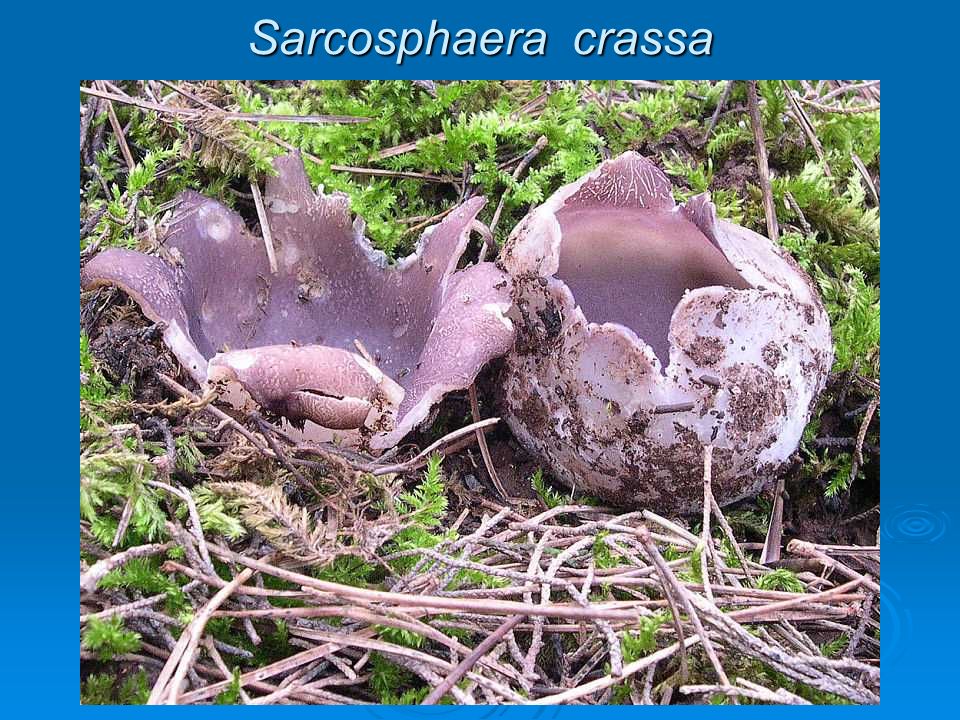The image depicts a detailed slide from a slideshow presentation. It features a thick border with a solid blue background, and in light blue letters at the top within the border, the title "Sarcosphaera Crassa" is prominently displayed. The central focus of the slide is a vivid, color photograph of a natural outdoor scene. The scene includes green leaves and brown twigs scattered on the ground. At the center, there is a distinctive, large, open shell-like structure, resembling two broken eggs or a cracked dinosaur shell. The shell has a white and brown-spotted exterior, with a solid brown interior that has lighter specks. The edges of the shell appear cracked and jagged. Accompanying the shell are two versions depicted on the right; both show the white and brown-spotted exterior with the solid brown interior visible, while the left side depicts a completely opened version of the shell. The setting is brightly lit with natural daylight, and the photo is taken against a backdrop of green foliage and dry, almost white grass-like stems, suggesting an outdoor, natural habitat.